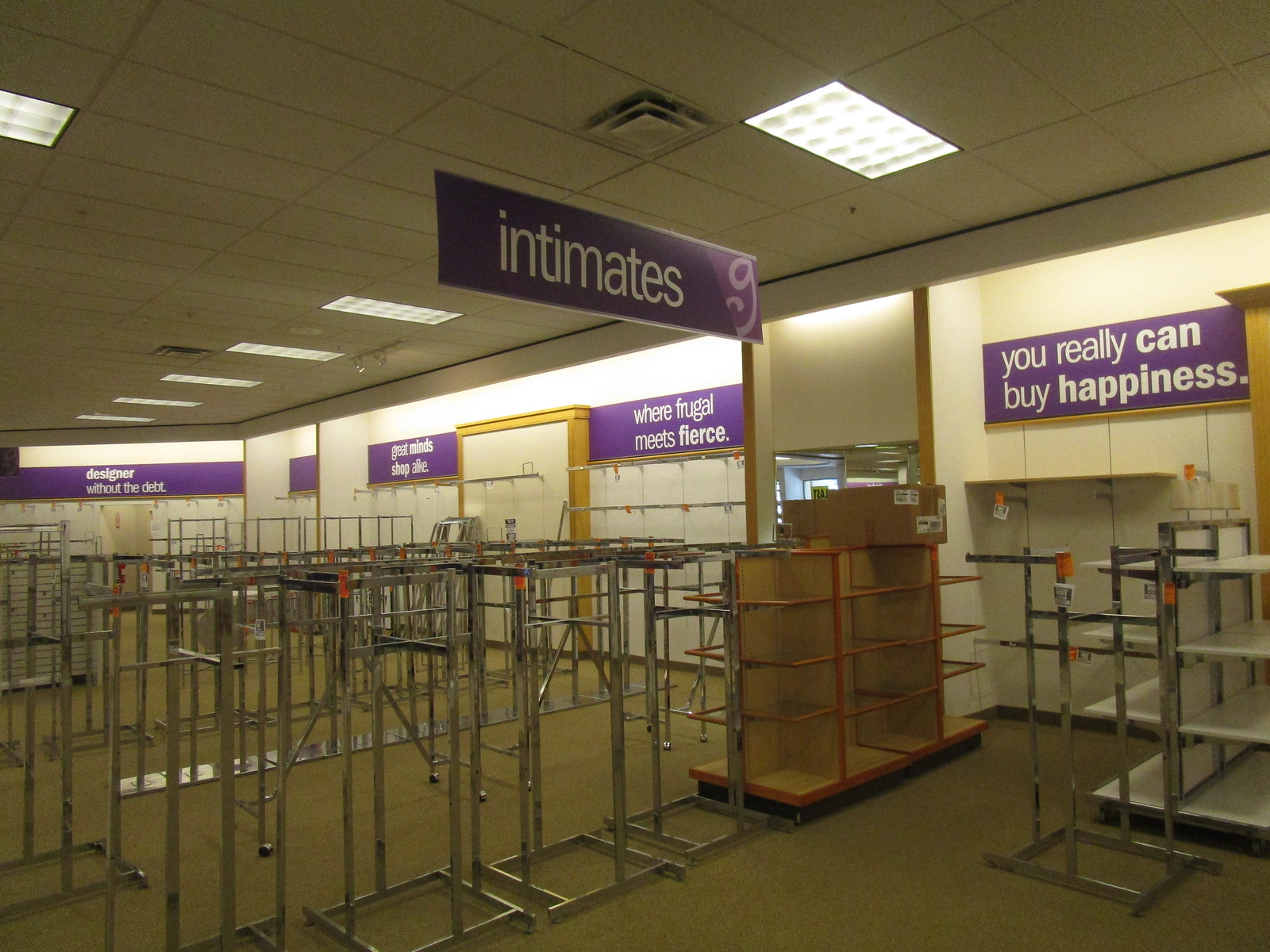This photograph captures the interior of a department store that appears to be in the midst of closing down or possibly preparing to open. The scene is characterized by barren racks meticulously arranged in rows, devoid of any merchandise. The store has a stark and minimalistic vibe, dominated by plain tile flooring and panel light ceilings, which contribute to the impersonal atmosphere. 

Several signs hang within the space, enhancing the narrative of the store's purpose. A prominent sign perpendicular to the wall reads "Intimates," indicating the section where undergarments are presumably sold or will be sold. Additional signs with a purple background and white font adorn the walls, featuring phrases like "You Can Buy Happiness," "Where Frugal Meets Fierce," and "Designer Without the Debt," highlighting the store's discount-oriented nature. These signs collectively convey a message of affordable luxury and budget-friendly shopping, underscoring the retail environment's focus on accessible fashion and value.